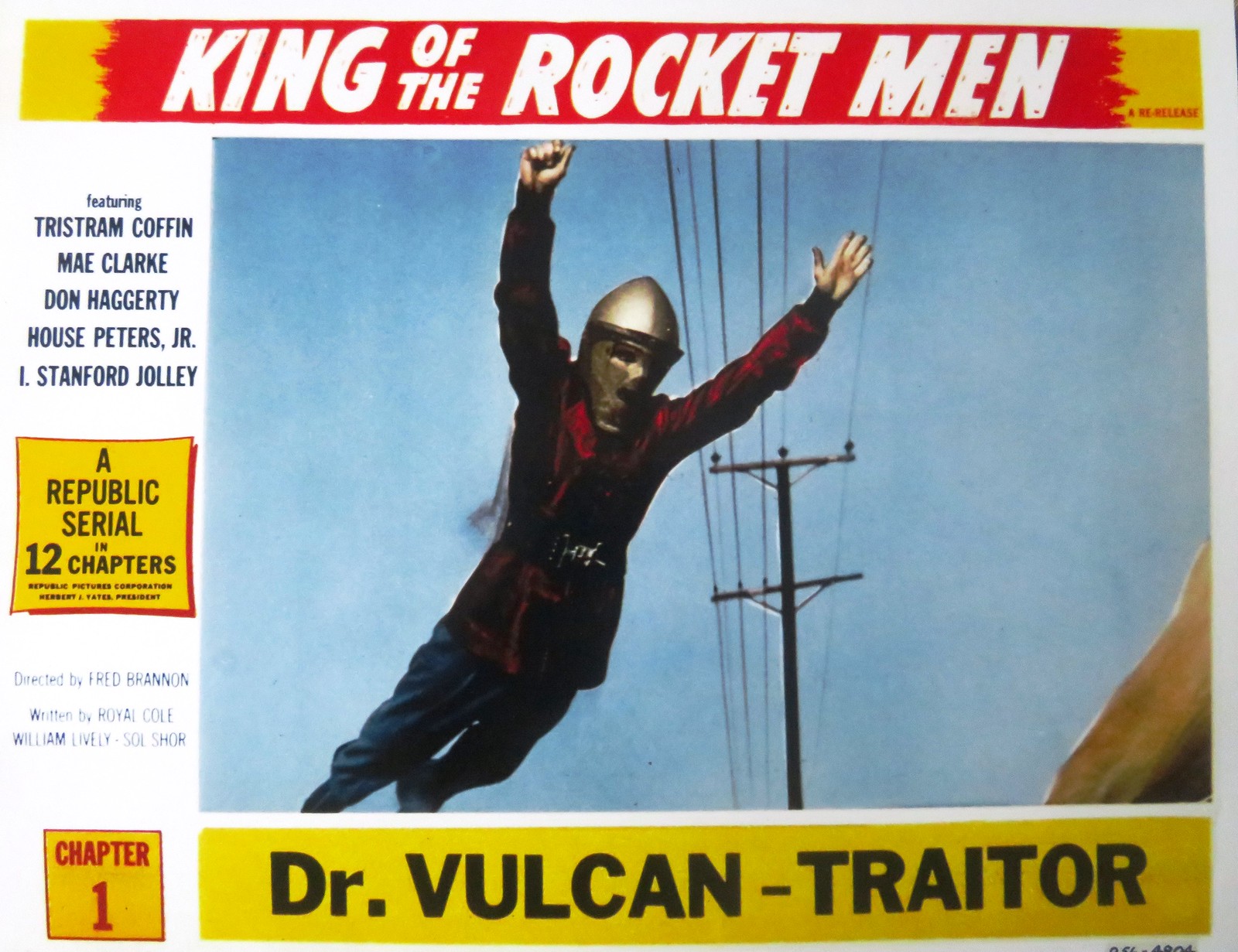The image is a vibrant advertisement for a classic TV show or movie serial titled "King of the Rocket Men." It prominently features a man in a dynamic pose, either flying or falling against a clear blue sky. He is equipped with a metallic, bullet-shaped helmet and wears a striking red suit with a long-sleeve, red and black tunic, along with a belt at the waist. His outfit appears to include darker boots and possibly baggy blue jeans. A jetpack is visible, strapped to his back, suggesting his airborne state. In the background, there's a telephone or utility pole with electric wires adding a touch of realism to the action scene.

At the top of the advertisement, a yellow and red banner boldly displays the title "King of the Rocket Men" in large white font. Below this, key information is presented: the series stars Tristan Coffin, Mae Clark, Don Haggerty, House Peter Sr., and J. I. Stantrick Jolly. The serial, directed by Fred Brennan and written by Royal Cole, William Lively, and SDR Shaw, consists of 12 thrilling chapters. The bottom section of the flyer, set against a yellow background with dark text, announces "Chapter 1, Dr. Vulcan Traitor", anchoring the audience's anticipation for an adventurous journey.